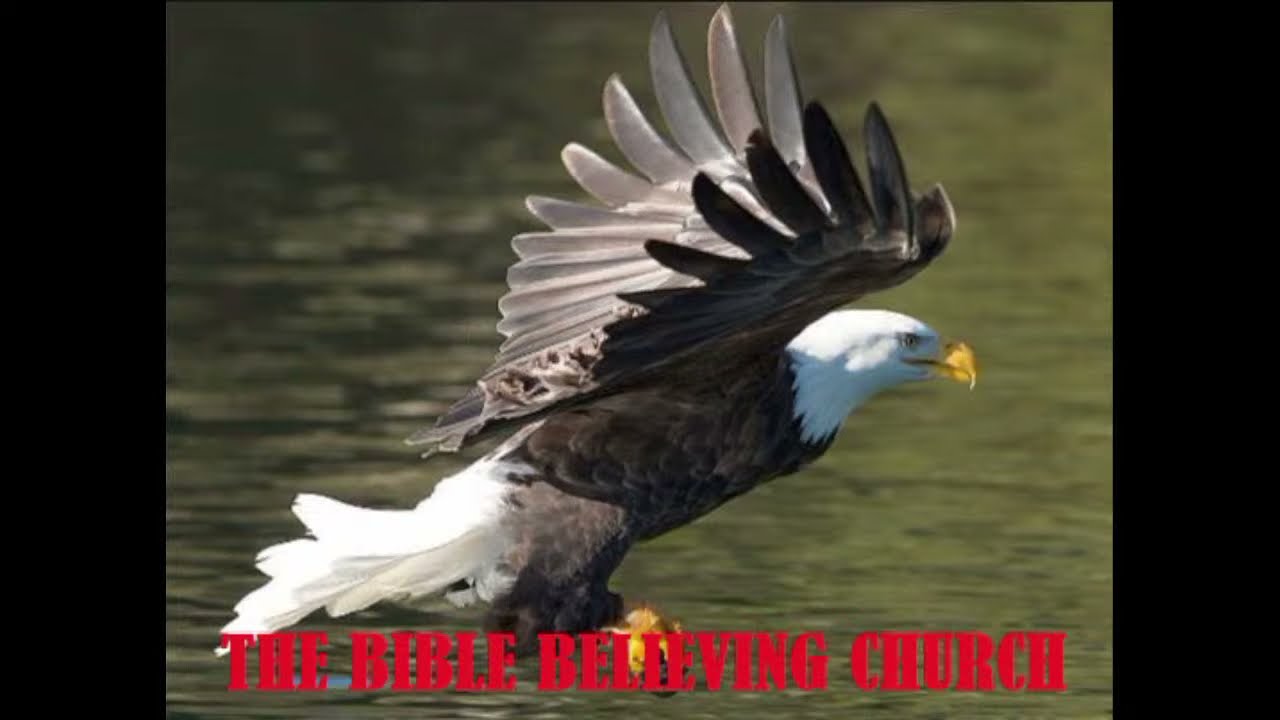The image depicts a majestic bald eagle in mid-flight, captured from the side in a profilic view. The eagle is soaring low over greenish-brown water, with the sunlight highlighting the top of its white head and body, while casting shadows on its underside. It has its wings fully spread, showing the contrasting white tail feathers against its dark gray or black wings. The eagle’s yellow beak and claws are prominently visible, indicating it might be about to snatch something from the water. At the bottom of the vibrant, daylight image, bold red capitalized letters spell out "The Bible Believing Church." The photo features a subtle black border on the left and right sides.